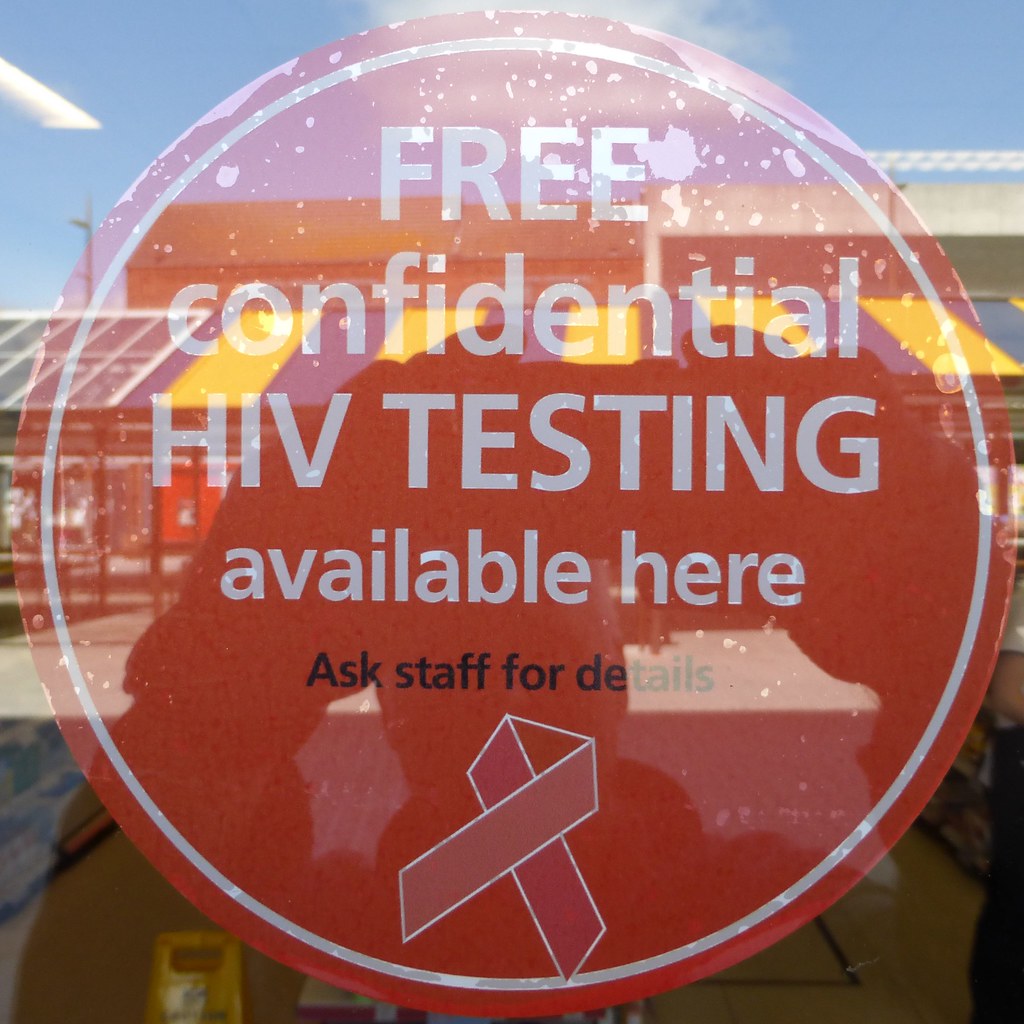The photograph is a square image showcasing a circular sticker on a window, likely of a business or medical office. The red sticker, bordered in white, prominently displays the message in bold white letters, "Free Confidential HIV Testing Available Here." Beneath this, in black text, it reads, "Ask Staff For Details." Below the text, there is a crisscross ribbon in various shades of pink and red. The photograph captures the reflection of the person taking the image, revealing their hands and the faint outline of their face, as well as a background featuring a striped yellow and blue pavilion-like structure. Outside the window, which suggests the sticker is placed on the inside of the glass, the glare indicates a bright, sunny day highlighted by blue skies and surrounding buildings.